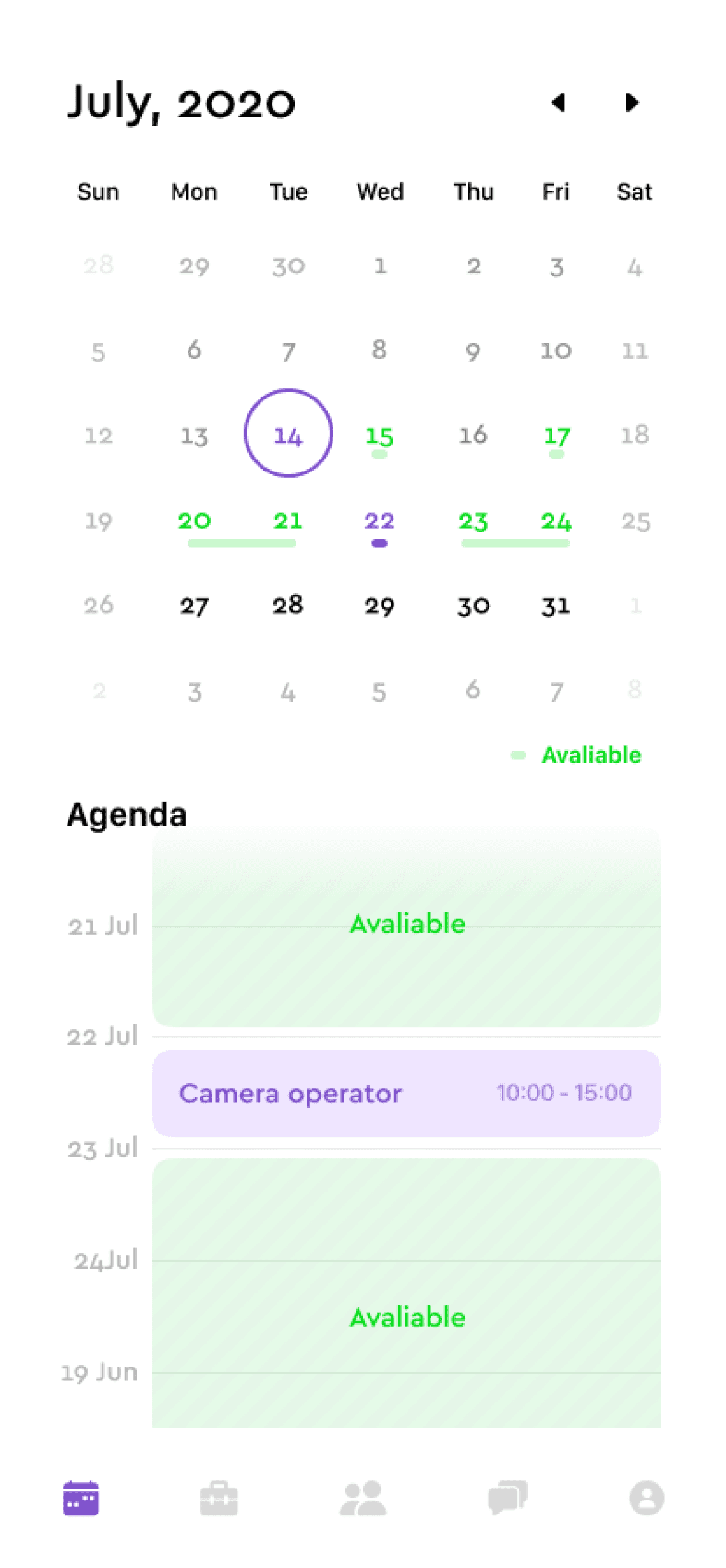In the image, a digital calendar for July 2020 is displayed. At the top, the header clearly shows "July 2020" with two navigation arrows on the right side; the left arrow is intended to navigate to previous months, while the right arrow allows navigation to upcoming months. Each day of the week is labeled: Sunday, Monday, Tuesday, Wednesday, Thursday, Friday, and Saturday. 

July begins on a Wednesday and concludes on Friday, the 31st. Key appointments are marked, including an agenda on the 31st, and "camera operator" scheduled on July 22nd from 10 a.m. to 3 p.m. Below the calendar, there are five icons, although their specific functions are not described in detail. 

The layout is structured and functional, providing easy navigation and a clear overview of monthly events and tasks.